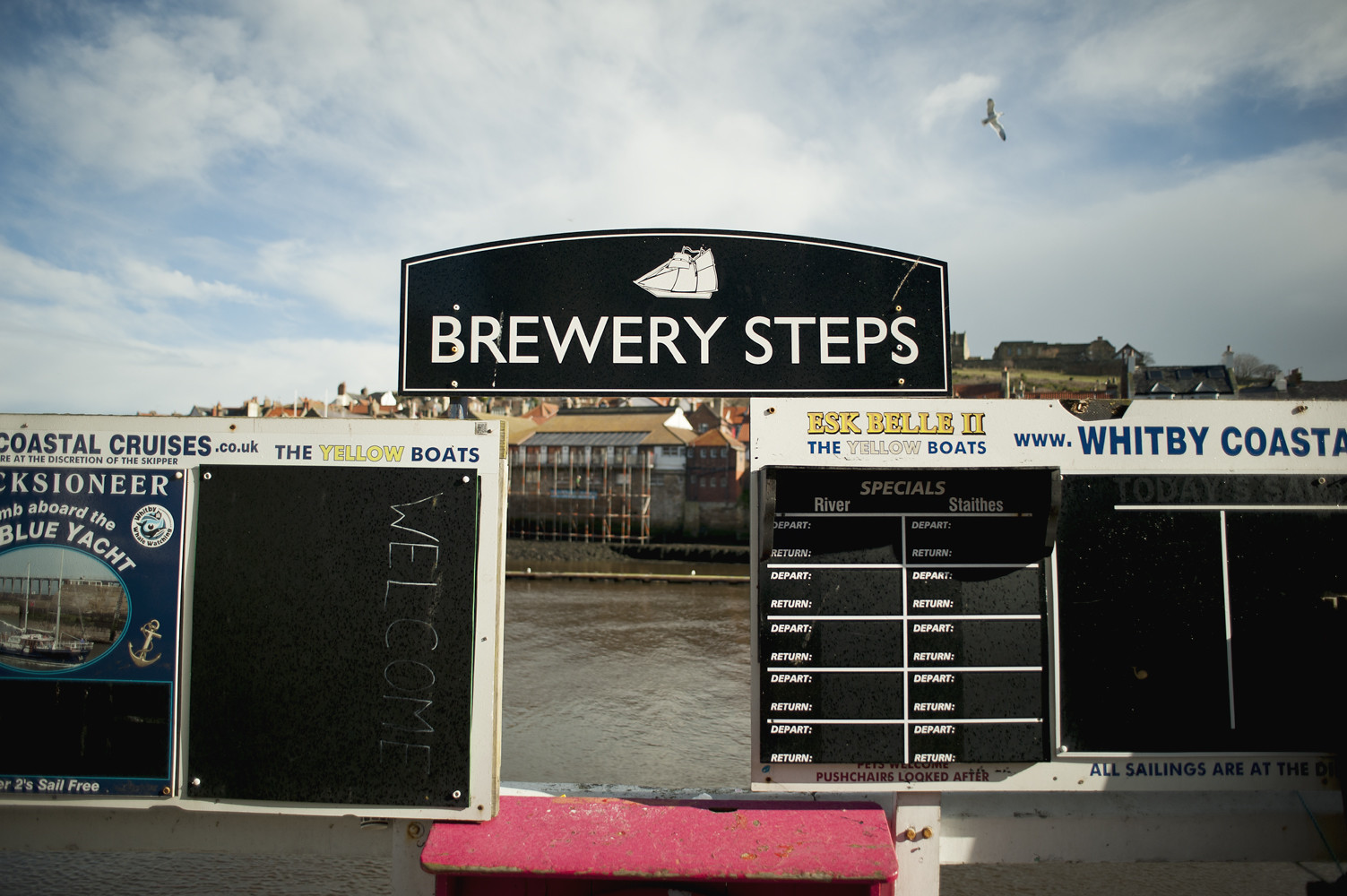This scene captures a vibrant riverside venue, characterized by a large, clean white wall adorned with several black chalkboards. Dominating the top of the chalkboards are small white banners advertising "ESK Belle 2" and "The Yellow Boats" from www.whitbycoastalcruises.co.uk. One prominent chalkboard, marked with the word "Welcome," sits vertically on the right side. To its left, an image of a blue yacht with the caption, "Sail Free," is prominently displayed. Another chalkboard lists departure and return times for boats, though it currently remains blank. Above these chalkboards, a sign reads "Brewery Steps," indicating a nearby area possibly designed for dining and watching boats. The scene reveals a vivid blue sky with a bird flying overhead, as well as a bustling town with dense architecture across the canal. Red painted steps with noticeable wear border the chalkboards, suggesting a historical charm to the venue. The glare from the sun adds to the authenticity of this lively waterfront setting.